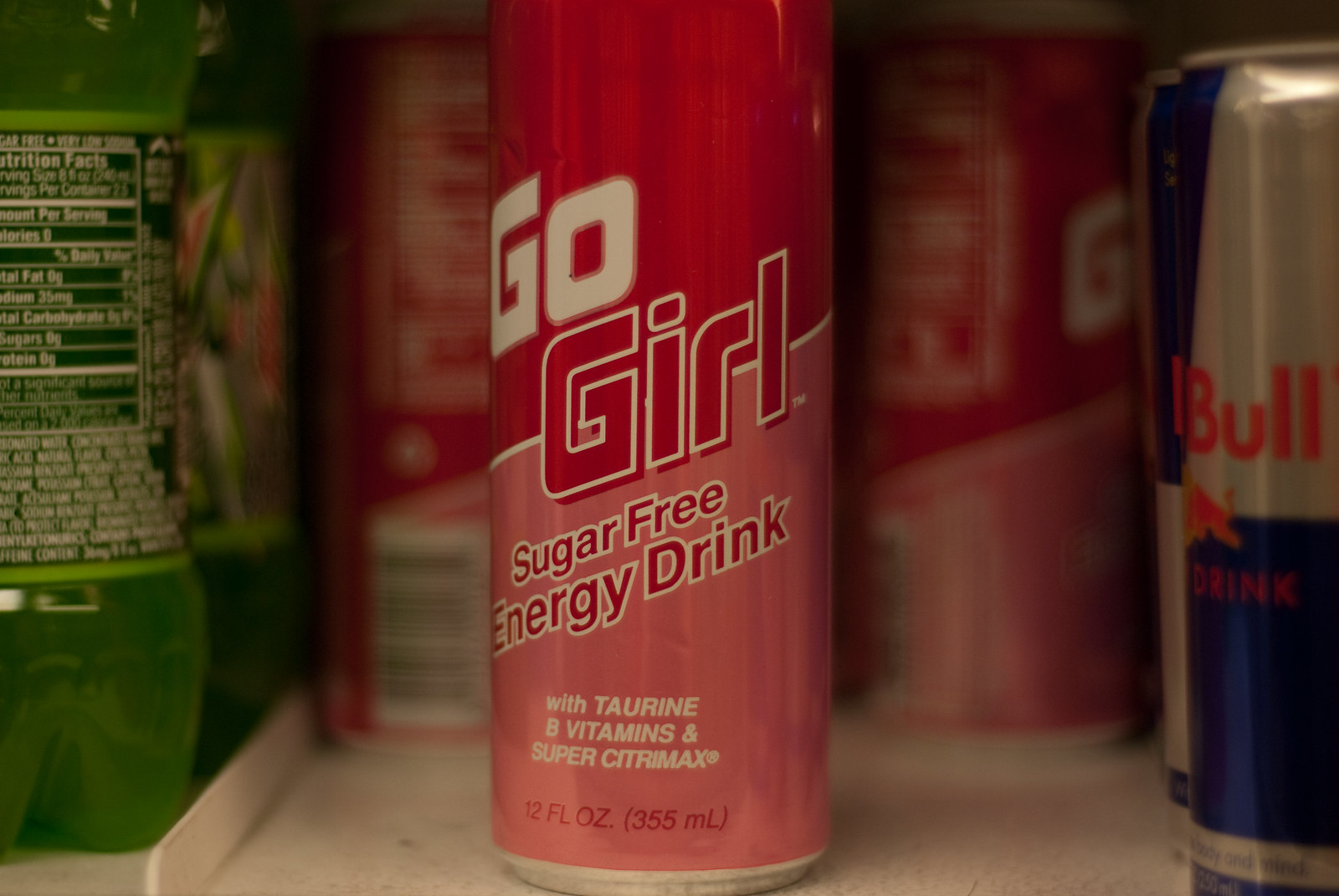In the center of the image is a prominently displayed can of "Go Girl" sugar-free energy drink. The can features a red top that transitions into a pinkish bottom, and it contains taurine, B vitamins, and Super CitriMax, with a label indicating 12 FL OZ (355 milliliters). In the background, slightly blurred, are additional cans and bottles. To the right, there are a couple of Red Bull cans, recognizable by their silver upper areas and blue lower sections, along with the distinctive red logo. On the left side of the image, two bottles of Mountain Dew are visible, showcasing the green soda inside and their nutrition facts labels.